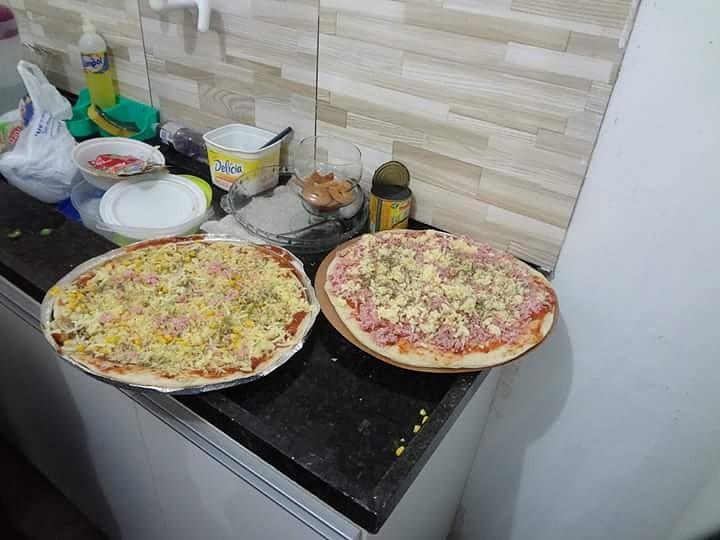The image depicts a slightly messy kitchen scene with two large, uncooked homemade pizzas occupying the black countertop. The pizza on the left, sitting on a silver lipped tray, features a thick layer of mozzarella cheese, pink meat pieces likely ham, and possibly some yellow corn. The pizza on the right, positioned on a round piece of cardboard, has a generous amount of pink meat and a thinner layer of cheese. Both pizzas are covered in red marinara sauce and await baking. Surrounding them are various empty containers, including an open can, a plastic tub with a "Delicia" butter label, plastic bags, a glass pie pan, a yellow bottle of dish detergent, and a yellow and green sponge. Crumbs and food waste are scattered across the countertop, which has a lip to prevent items from sliding off. The backsplash features a faux beige wood effect, contrasting with plain white walls farther to the right. Overall, the kitchen exhibits an unclean, cluttered setup, suggesting someone has just finished preparing the pizzas.